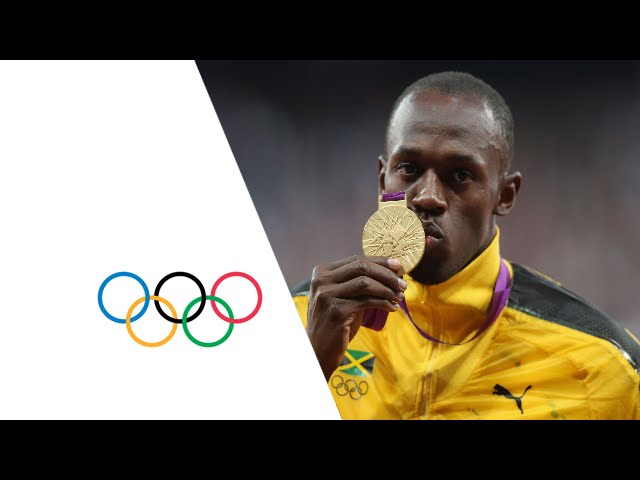This image is a poster advertising the Olympics featuring a black male Olympian holding and kissing a gold medal. The poster is divided with a distinctive design: on the left side, a white diagonal stripe narrows as it ascends from a wider base at the bottom, bordered by black frames at the top and bottom. Within this white stripe, the iconic Olympic rings, in blue, yellow, black, green, and red, are prominently displayed. On the right side of the image stands the Olympian against a gray background. He sports a yellow tracksuit with black detailing on the epaulets, a Jamaican flag on his right breast, below which is the Olympic logo, and the Puma logo on his left breast. The gold medal, hanging from a purple ribbon, is in his left hand, which he is kissing.